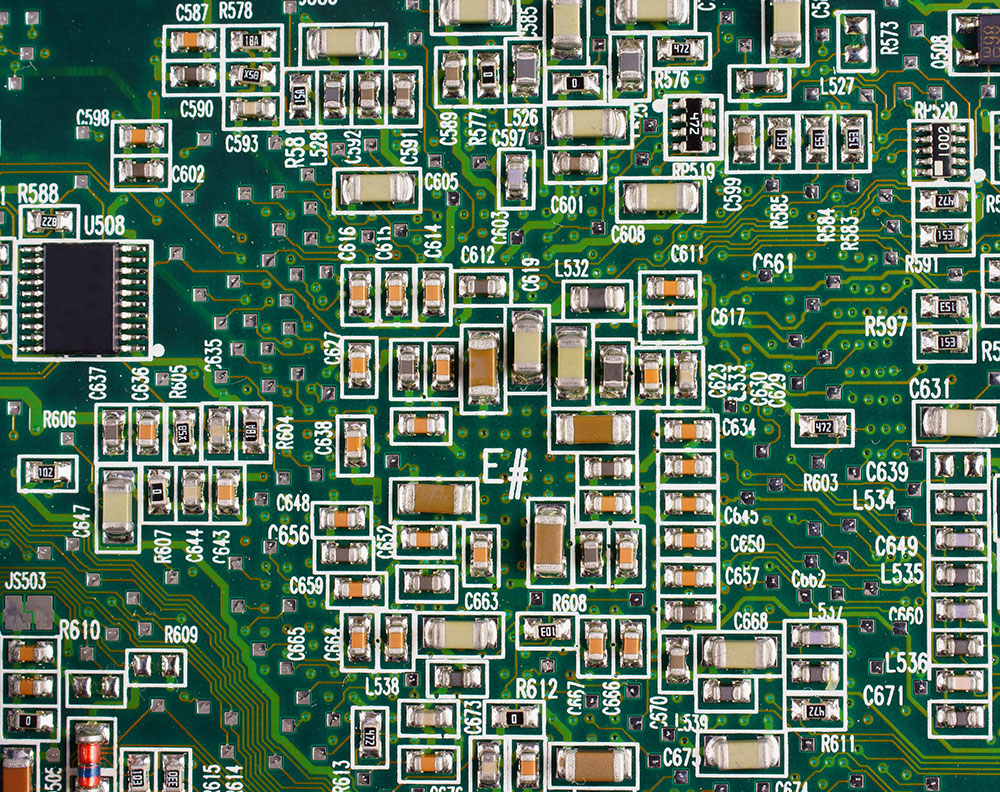The image displays a detailed close-up of a square green circuit board, adorned with numerous small beige and brown capacitors, each featuring metallic gray ends. The green background exhibits a mixture of dark and olive green hues, with a solid dark brown area in the upper left and olive green zigzag lines in the lower left corner. Scattered across the board, these capacitors are marked with numbers and letters, many beginning with C, L, or R, such as C671 in the lower right corner. Towards the upper part of the left side, there is a larger black square component, outlined in white with horizontal dashes on its sides, labeled U508. This intricate array of components, with metallic traces possibly made of copper or gold interconnecting them, creates a highly technical and complex appearance typical of a silicon-based circuit board.